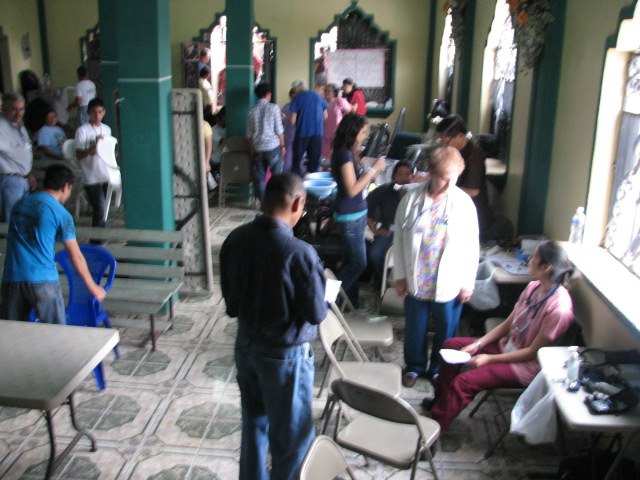This image portrays a bustling makeshift medical clinic, possibly situated in South America or a Caribbean island. The setting is an interior room filled with approximately 15 people, some seated and others standing, dispersed throughout the space. Dominating the color palette of the room are vibrant hues worn by the people, including whites, pinks, blues, and reds. The chairs and benches are in shades of gray, tan, and blue, complementing the blue, white, and green-tiled floor. 

On the right side, two women, seemingly medical professionals, wear pink scrubs and a white coat with stethoscopes around their necks. One, in pink scrubs and blue pants, is engaged in conversation with the woman in the white coat adorned with a floral shirt and blue pants. To the left, a man stands facing away from the camera in a blue shirt and jeans. The walls are a tan or yellow hue, and the room's structural details include three greenish-blue support beams on the top left and mirrored elements on the back wall.

The overall scene is lively, with individuals moving and interacting in what appears to be an active environment dedicated to medical evaluations. The architectural elements, such as the scalloped triangular tops of the windows, enhance the room's local, possibly tropical, aesthetic.